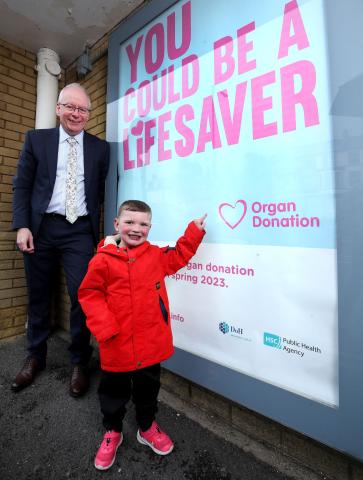This vibrant color photograph captures a joyous moment between an older gentleman and a young boy. Set against the side of a brick building, the scene is marked by a large advertisement encased in a gray frame with a plastic cover. The advertisement prominently features bold pink letters reading, "You could be a lifesaver. Organ donation," accompanied by a heart symbol. Notably, the boy, who appears to be around six or seven years old, has short brownish hair with a reddish tint, and he is dressed in black pants, red shoes, and a striking red coat. He stands in front, pointing enthusiastically at the sign, his face beaming with happiness as he directly engages the camera.

Behind the boy stands an older man — possibly the boy's grandfather or doctor — exuding a warm, proud smile. He sports a dark blue suit, a white shirt, and a beige-yellow patterned tie. His white hair is thinning, and he wears glasses, adding a touch of wisdom to his appearance. The duo stands on a dirt-covered macadam surface, reinforcing the outdoor setting of the photograph. The entire scene suggests a moment of shared pride and joy, perhaps indicating the boy's life was saved by an organ donation, celebrating the impactful message displayed on the sign.